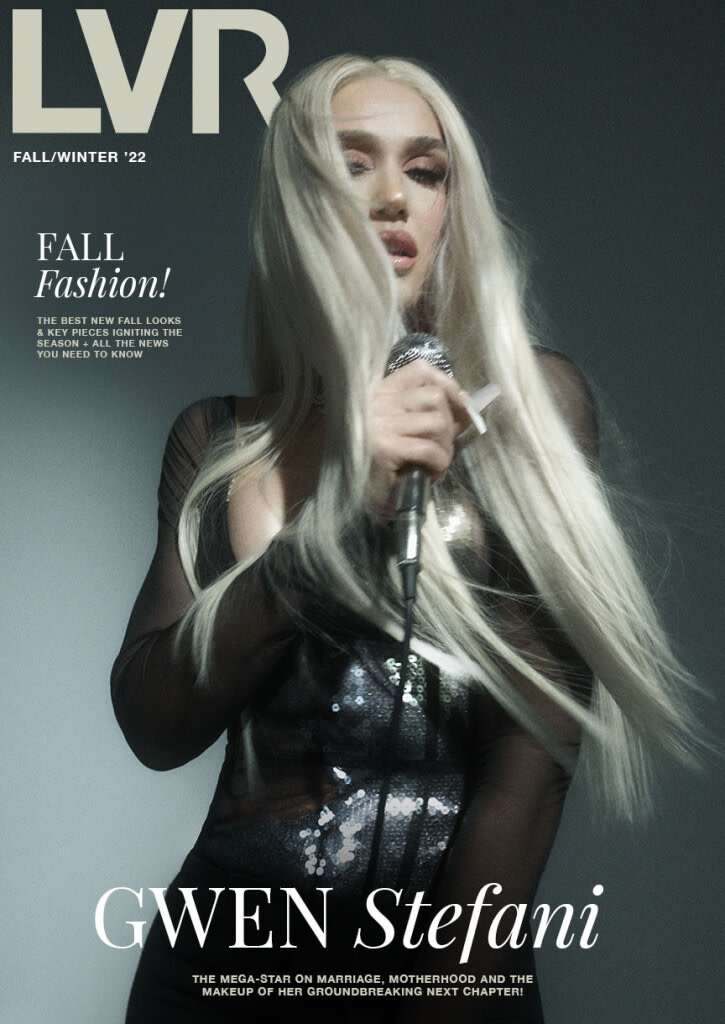The cover of the fall-winter 2022 edition of LVR magazine features Gwen Stefani centered against a deep, grayish-green background. Her name is prominently displayed in two different fonts, "Gwen" in one and "Stefani" in another. Stefani's platinum blonde hair, cascading to mid-waist, is dramatically blowing into her face and over her body. She wears a striking black and silver sequined dress with sheer, low-cut sleeves, though her modesty is maintained by the microphone she holds in her right hand, with her left by her side. Her heavy eye makeup and full pink lips are accentuated by her long, rounded white nails. At the bottom, a byline highlights her story on marriage, motherhood, and her groundbreaking next chapter. To her left, the words "Fall Fashion" in matching font colors discuss the best new fall looks, key pieces igniting the season, and essential news, all emphasized by the print matching Stefani’s striking hair color, making the text pop against the dark background.